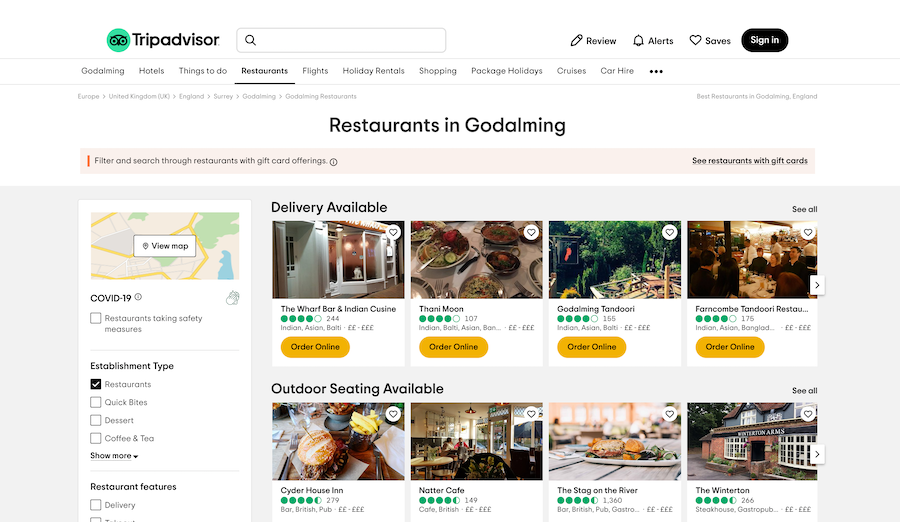The image features a TripAdvisor web page prominently displayed. At the top left corner, the TripAdvisor logo is visible, rendered with green and black colors and featuring a stylized owl face. To the right of the logo, there's a search bar followed by a row of tabs labeled: "Review," "Alerts," "Saves," and "Sign In," with the "Sign In" button highlighted in black.

Directly below this section lies another navigation menu, starting with the options "Go aiming," "Hotels," "Things to Do," "Restaurants," "Flights," "Holiday Rentals," "Shopping," "Package Holidays," "Cruises," "Car Hire," and an additional options menu represented by three dots.

The page headline reads "Restaurants in God aiming," followed by a subheading on a pink background, offering information and a call-to-action: "Filter and search through restaurants with gift card options. See restaurants with gift cards."

Further down the page, restaurants are categorized into two main sections: those with "Delivery Available" and those with "Outdoor Seating Available." On the left sidebar, there is a menu featuring options like "Map," "COVID-19," and several checkboxes for filtering results by categories such as "Establishment Type," "Restaurant," "Quick Bites," "Dessert," and "Coffee & Tea."